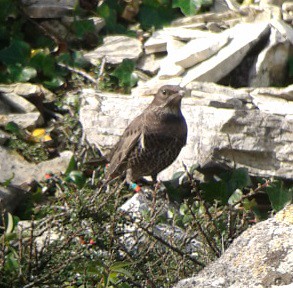This photograph is a square, clear, and naturally-lit image featuring a medium-sized bird, resembling a pigeon, perched on a log amidst a grassy area with scattered rocks and bushes. The bird, facing slightly to the right, is adorned in varying shades of dark gray, brown, and some hints of white, particularly on its small beak. A distinguishable feature is the band on its front right leg, colored turquoise and orange, indicative of tracking or tagging. The backdrop showcases a natural setting with different sized rocks, logs, and patches of grass and dirt, highlighting the bird as the focal point.